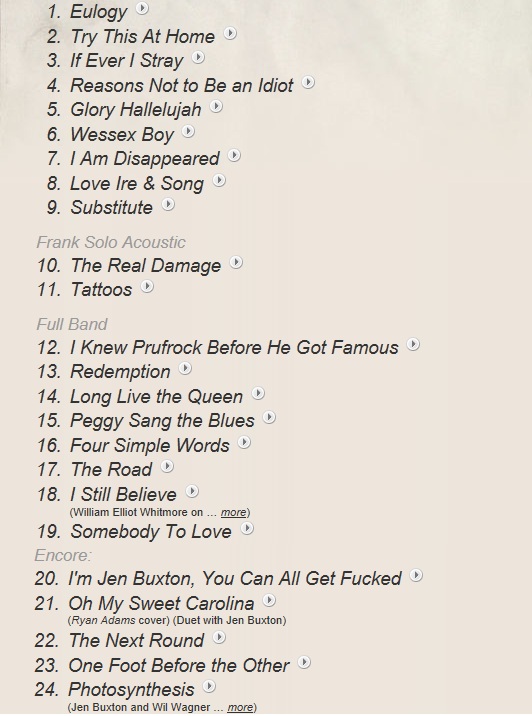The image is a portrait-oriented printed publication featuring a detailed, numbered list of 24 song titles. The background is a light beige or off-white color, and the text is printed in black, italic, upper and lowercase. The songs are listed from top to bottom, aligned on the left side. The first section includes numbers 1 through 9: "Eulogy," "Try This at Home," "If Ever I Stray," "Reasons Not to Be an Idiot," "Glory Hallelujah," "Wessex Boy," "I Am Disappeared," "Love, Ire, and Song," and "Substitute." 

Following this, there's a section titled "Frank Solo Acoustic" in light gray, featuring songs 10 and 11: "The Real Damage" and "Tattoos." Another heading in gray, "Full Band," introduces items 12 through 19: "I Knew Prufrock Before He Got Famous," "Redemption," "Long Live the Queen," "Peggy Sang the Blues," "Four Simple Words," "The Road," "I Still Believe" (with "William Elliot Whitmore" noted underneath), and "Somebody to Love." 

A final section labeled "Encore" in light gray includes numbers 20 through 24: "I'm Jen Buxton, You Can All Get Fucked," "Oh My Sweet Carolina" (noted as a Ryan Adams cover and duet with Jen Buxton), "The Next Round," "One Foot Before the Other," and "Photosynthesis" (featuring Jen Buxton and Will Wagner).